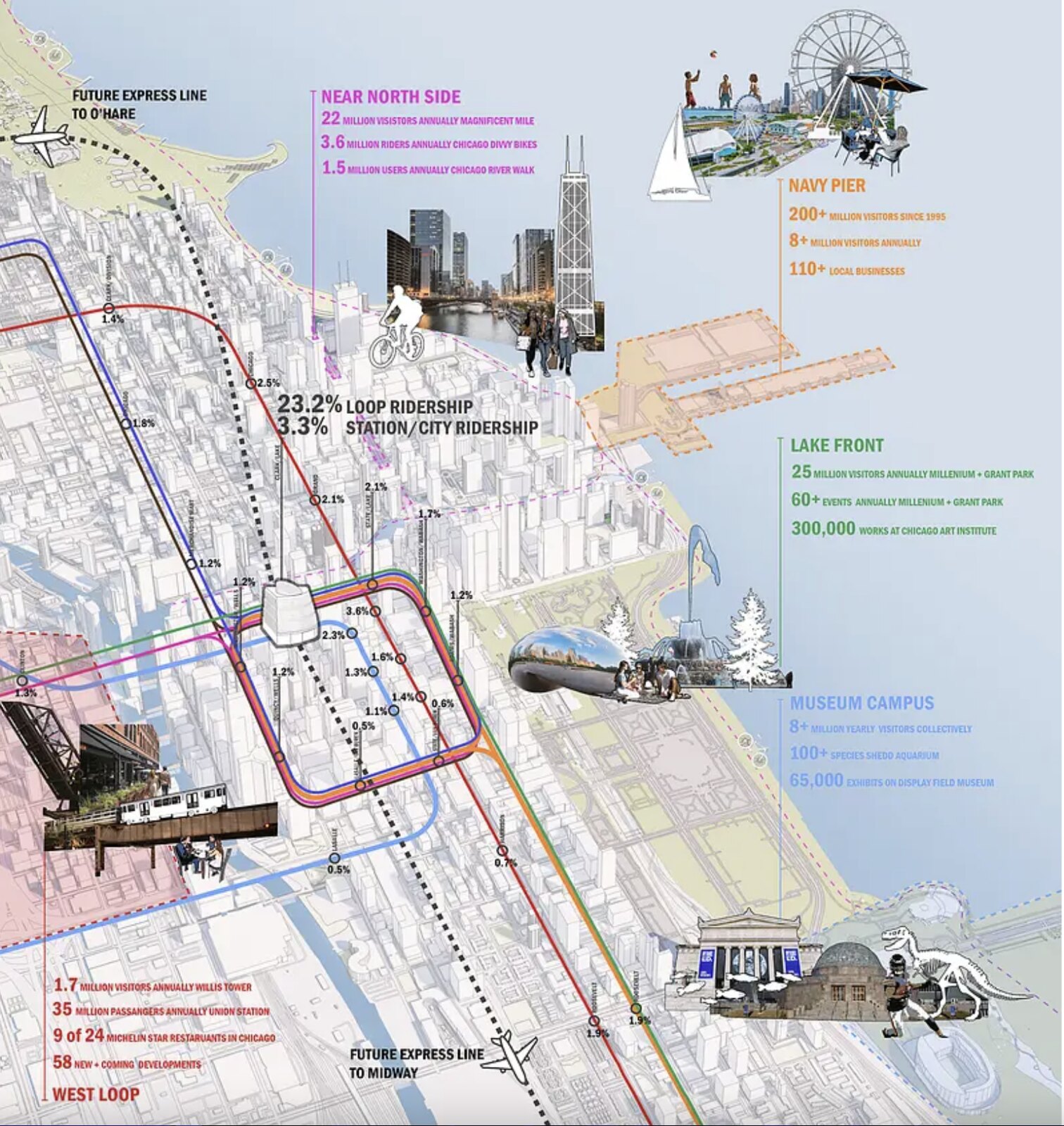The image is an infographic presented as an aerial map of Chicago, emphasizing various landmarks and transportation routes. The background consists of a faint city overview with distinct colorful lines representing different transit paths: green, yellow, red, pink, and blue. At the top left corner, a little airplane icon with a dotted line connecting it to the center indicates a "Future Express Line to O'Hare." Similarly, at the bottom, another airplane icon denotes a "Future Express Line to Midway."

Key landmarks and statistics are strategically placed around the map. The upper right features Navy Pier with details such as "200+ million visitors since 1995" and "110+ local businesses" highlighted in orange. Adjacent to this is an area showcasing people engaged in activities like playing volleyball and sailing, underscored by attractions such as the Ferris wheel. Nearby, highlighted in pink, are points of interest like the Near North Side, which boasts "22 million visitors annually" and "3.6 million riders annually" on the Magnificent Mile.

The map also highlights the Lakefront area in green, emphasizing "25 million visitors annually" and key locations like Millennium and Grant Park with "60+ events annually" and "300,000 works" at the Chicago Art Institute. Moving downward to the Museum Campus section, depicted in blue, it mentions "8+ million yearly visitors collectively" and notable attractions like the Shedd Aquarium and Field Museum.

Towards the lower left, a section marked in red details the West Loop with significant figures such as "1.7 million visitors annually" at Willis Tower and "35 million passengers annually" at Union Station. In the map's center, statistical figures display transportation hub data with "23.2% Loop Ridership" and "3.3% Station City Ridership."

The infographic uses a color palette featuring light blue, pink, orange, green, red, yellow, white, and black to differentiate various elements and bring attention to Chicago's bustling activity centers and transportation network.